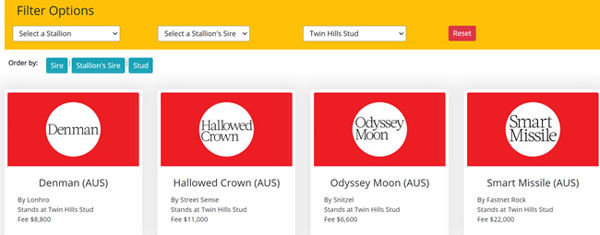This image is a screenshot from an unidentified application or website, featuring a filtering and sorting interface for selecting stallions and their sires. At the top, a dark yellow bar contains several filter options with accompanying drop-down arrows labeled "Select a Stallion," "Select a Stallion Sire," "Twin Hills Stud," and a "Reset" button.

Below this bar, the background transitions to white and presents sorting options labeled "Order by Sire," "Stallion Sire," and "Stud." The main content area showcases four distinct entries for stallions, each within a red square containing a white circle with the name of the stallion in bold:

1. **Denman**
   - **Details:** Denman (AUS), sired by Lonhro, currently stands at Twin Hills Stud with a fee of $8,800.
   
2. **Hallowed Crown**
   - **Details:** Hallowed Crown (AUS), sired by Street Sense, currently stands at Twin Hills Stud with a fee of $11,000.
   
3. **Odyssey Moon**
   - **Details:** Odyssey Moon (AUS), sired by Snitzel, currently stands at Twin Hills Stud with a fee of $6,600.
   
4. **Smart Missile**
   - **Details:** Smart Missile (AUS), sired by Fastnet Rock, currently stands at Twin Hills Stud with a fee of $22,000.

The image is oriented in landscape format, being wider than it is tall.